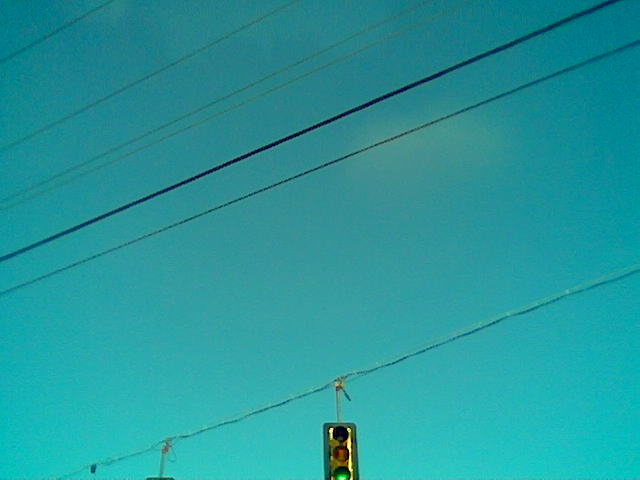In the image, a bright blue sky with wisps of clouds forms the backdrop for a complex network of electrical wires and cables, with six or seven distinct lines diagonally crossing the frame from the upper left. These lines vary in thickness, with one notably thicker black wire among the lighter ones. At the bottom of the image, a standard traffic light, encased in yellow with a dark green or black border, hangs suspended from a smaller wire attached to the main cables. The visible light is shining green, indicating that it’s currently set for go. Nearby, a second traffic light is partially visible with only its top edge peeking into the frame.